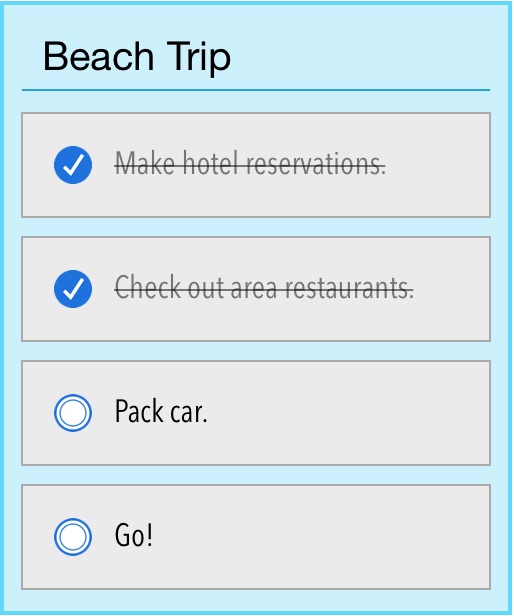The image shows a vibrant, blue background with a neatly organized checklist in gray boxes. Items on the list such as "Make hotel reservation" and "Check out area restaurants" are marked with check marks and crossed out, indicating they have been completed. Next items on the list, including "Pack car" and "Go," have circles beside them, suggesting they are pending tasks. Below the checklist, a peculiar pricing chart lists costs uniformly at $1.00, regardless of the number of people, ranging from 1 to 15. The scene concludes with a courteous "Thank you for watching!" message, creating a welcoming and informative visual layout.